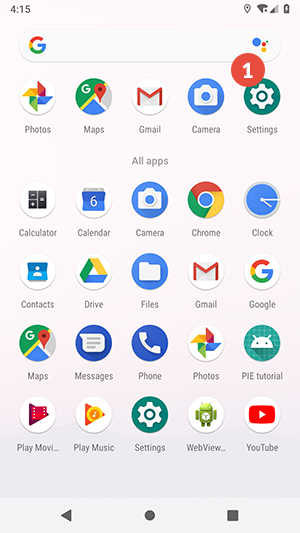Detailed Caption:

The image showcases an Android smartphone's interface displaying a variety of app icons on the home screen. At the top of the screen, the time is clearly indicated as 4:15 PM. Adjacent to the time, the upper right corner contains several status icons. Located just below this information is a prominently featured Google search bar. 

Beneath the search bar, a grid of app icons is visible. The icons include Photos, Maps, Gmail, Camera, and Settings, among others. A noticeable feature is a red notification badge with the number '1' overlaying the Settings icon, indicating there is one notification related to the settings.

Further down, another section labeled "All Apps" is present, listing apps like Calculator, Calendar, Camera, Chrome, Clock, Contacts, Drive, Files, Gmail, Google, Maps, Messages, Phone, Photos, PIE, Tutorial, Play Movies (though the entire word "Movies" is partially cut off), Play Music, Settings, WebView (partially visible as "WebView..."), and YouTube. Each of these apps is represented by circular icons featuring distinct logos or symbols within them.

At the very bottom of the screen, there are navigation buttons consisting of a dot centered in the middle, an arrow pointing to the left, and a square on the right-hand side, which are standard interface elements for Android devices.